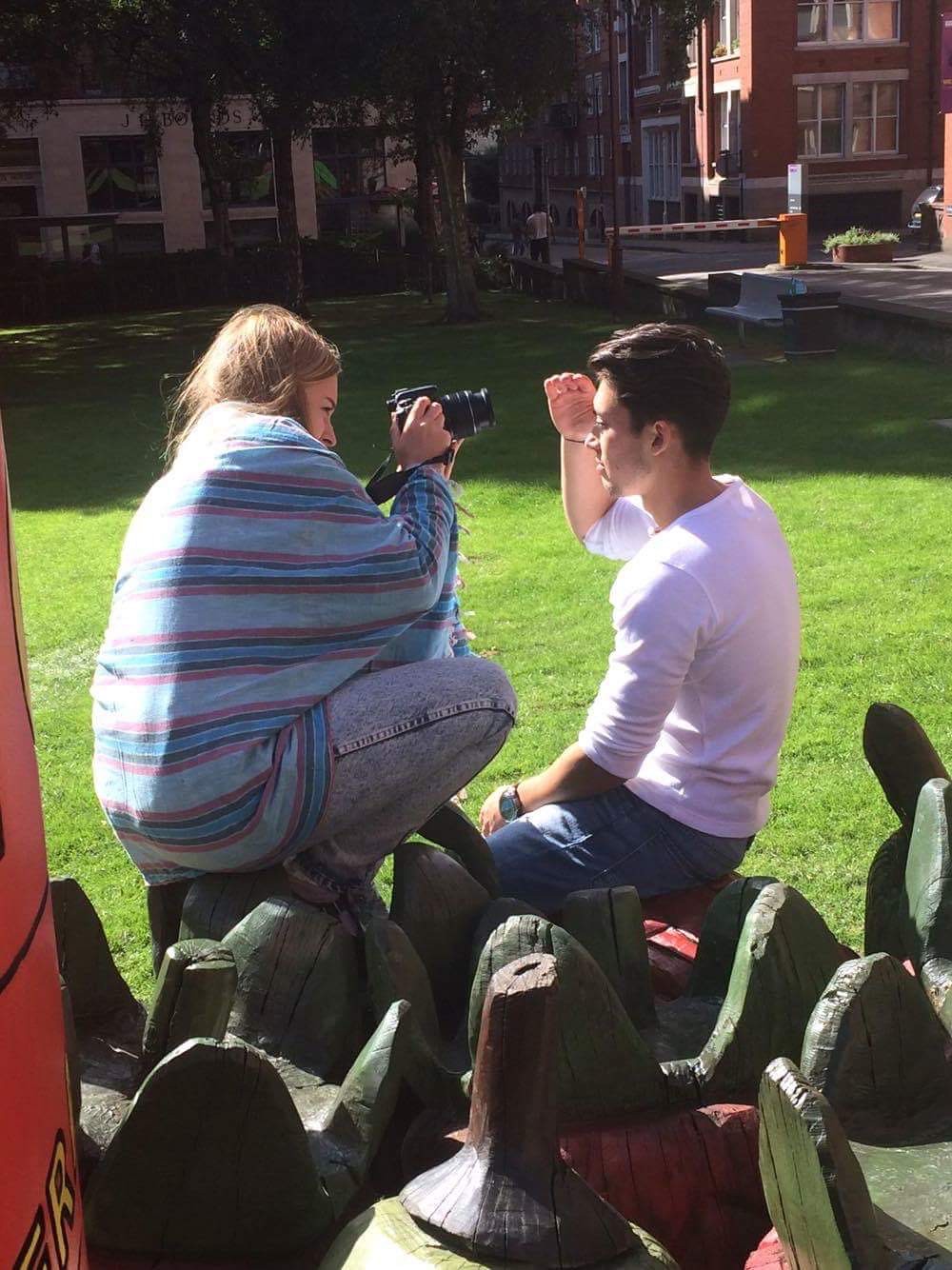In this vibrant outdoor scene, a young white female on the left is intently focused on capturing a photograph with her professional DSLR camera. Positioned on a wooden structure that could be part of a public art installation, she is photographing a person on the right who appears to be male, though his race is ambiguous. Both individuals are seated on the wooden structure, which is set in the middle of a lush green field. In the background, two historic buildings add a touch of antiquity to the setting, along with a visible parking lot. The brilliant sunlight illuminates the male's face and casts a radiant glow on the female's back, highlighting the bright, clear day.